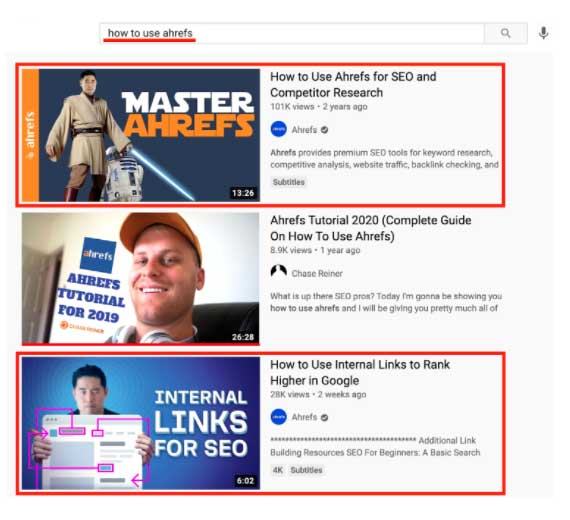This image is a screenshot of search results, presumably from YouTube or Google, based on the presentation of the results. The search query entered is "how to use Ahrefs," with the query text underlined in red, added later to the screenshot. At the end of the search bar, there's a search button represented by a magnifying glass icon, and adjacent to it, outside the search bar, is a microphone icon.

The search results consist of three video thumbnails, each containing associated information. Both the first and last video thumbnails are circled in red, suggesting they are desirable results.

1. **First Video:**
   - **Thumbnail Description:** A man resembling a Jedi character with R2-D2 in the background at his left. The man is facing towards the right side of the image (his left).
   - **Title:** "Master Ahrefs"
   - **Video Information:** The title reads "How to Use Ahrefs for SEO and Competitor Research." It includes the number of views, the upload date, user details, and a brief description.

2. **Second Video:**
   - **Thumbnail Description:** A man facing left, wearing a baseball cap and headphones around his neck.
   - **Title:** "Ahrefs Tutorial for 2019"
   - **Video Information:** Despite the thumbnail title, the video description reads "Ahrefs Tutorial 2020, Complete Guide on How to Use Ahrefs." It also includes the number of views, the upload date, user details, and a brief description.

3. **Third Video:**
   - **Thumbnail Description:** An Asian man holding a large piece of paper with various highlights in purple, standing against a blue background that graduates from dark to light blue.
   - **Title:** "Internal Links for SEO"
   - **Video Information:** The headline states "How to Use Internal Links to Rank Higher in Google." Similar to the other entries, it includes the number of views, the upload date, user details, and a brief description.

Overall, the red circles and underlines in the screenshot appear to emphasize important elements and guide viewers' attention to specific results and search terms.